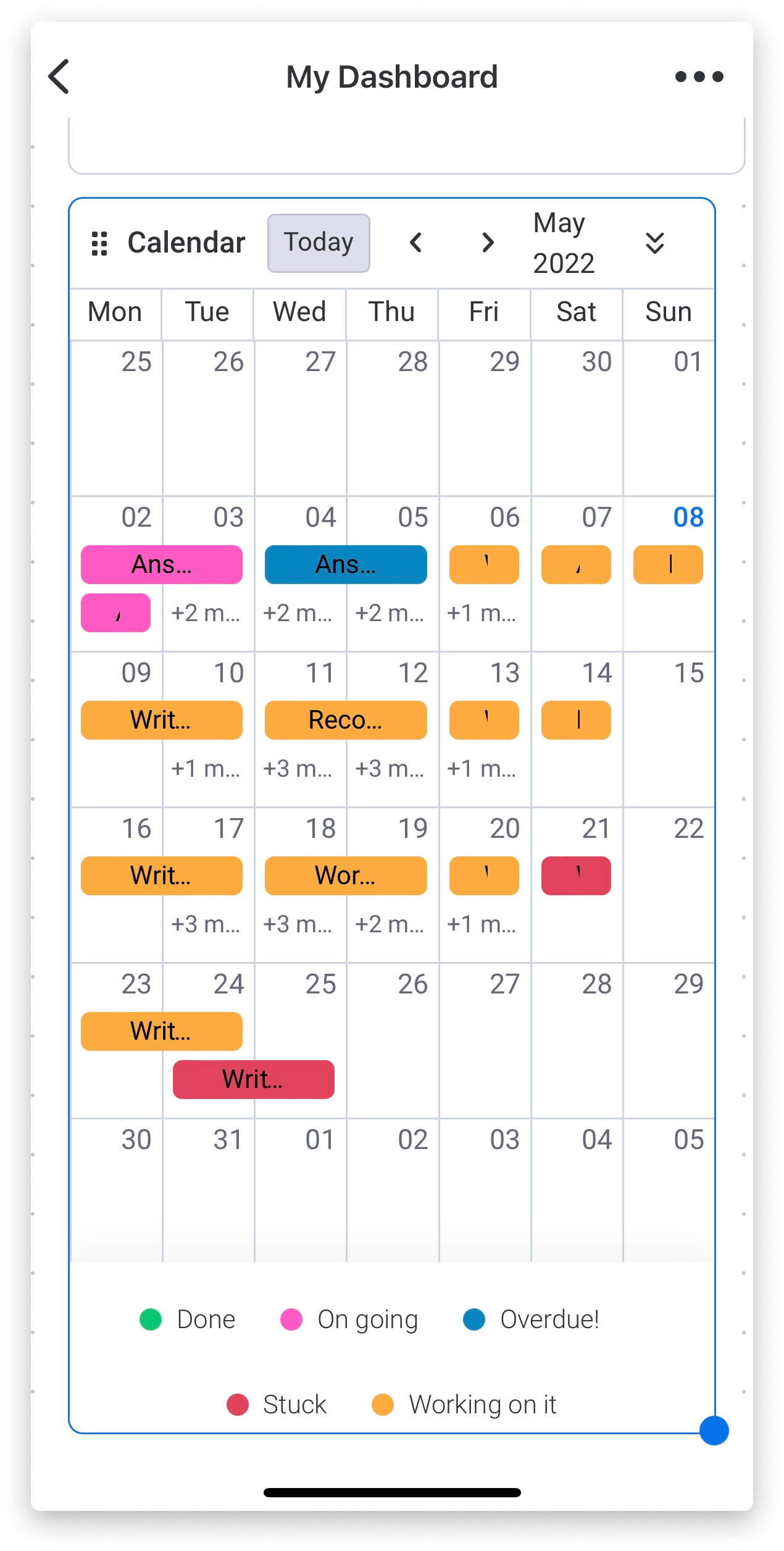This image is a detailed screenshot of a personal dashboard interface. The layout is vertically rectangular with an all-white background. At the top, there is a left-pointing black arrow icon, indicating a navigation element. Centrally aligned at the top is the title "My Dashboard," written with capital letters for 'M' and 'D.' On the right side of the title, there are three horizontally aligned dots which typically indicate additional options or settings.

Below this header section, there is a segmented area with a blue outline. Inside this segment, there are two columns of vertically arranged, evenly spaced triple dots (similar to a menu icon), divided into three rows with each row containing two dots.

To the right, there is a section titled "Calendar," with 'C' capitalized, set against a gray background with the word "Today" prominently displayed in the same style. Flanking the calendar's title are left and right arrows, likely for navigation through different dates.

The current month displayed is "May 2022," accompanied by a double downward arrow suggesting a dropdown menu for month selection. The days of the week are abbreviated to three-letter forms: "Mon," "Tue," "Wed," "Thu," "Fri," "Sat," and "Sun." Each day header is followed by a column of dates listed in order. 

For example:
- Under "Mon": 25, 02, 09, 16, 23, 30.
- Under "Tue": 26, 03, 10, 17, 24, 31.
- Under "Wed": 27, 04, 11, 18, 25, 01.
- Under "Thu": 28, 05, 12, 19, 26, 02.
- Under "Fri": 29, 06, 13, 20, 27, 03.
- Under "Sat": 30, 07, 14, 21, 28, 04.
- Under "Sun": 01, 08 (highlighted in blue), 15, 22, 29.

At the bottom of the screenshot, there is a legend explaining different colored circles with status labels:
- Green Circle: "Done"
- Pink Circle: "Ongoing"
- Blue Circle: "Overdue" (accompanied by a question mark or exclamation point symbol)
- Red Circle: "Stuck"
- Orange-Yellow Circle: "Working on it"

This interface appears to be a task management or scheduling application, visually structured to offer users an intuitive summary and navigation of their daily and monthly tasks.